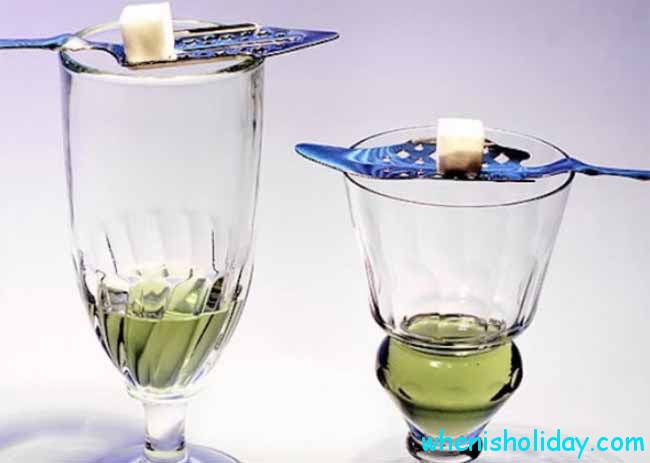In the image, there are two clear crystal glasses positioned against a white background, possibly on a white table, with a shadow cast to the left. The taller glass on the left is a goblet-style wine glass with a swirl design and is about 25 percent full of green liquid. The shorter glass on the right is a miniature goblet with a curvaceous, ball-shaped bottom, also containing about 25 percent green liquid. Each glass has a blue, flat spatula with diamond-shaped holes resting on top, and atop each spatula sits a white cube, possibly a sugar cube. The website name "whenisholiday.com" appears in the bottom right corner in a light teal blue, Comic Sans-type font.